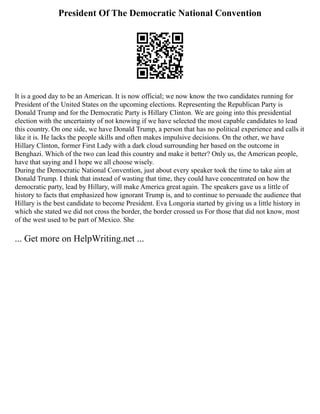The image is a scanned document titled "President of the Democratic National Convention," prominently featuring a black and white QR code. The main body of text highlights the official announcement of the 2016 U.S. presidential candidates: Donald Trump representing the Republican Party and Hillary Clinton for the Democratic Party. The text expresses the nation's uncertainty about the candidates' capabilities, questioning Trump's political inexperience and impulsivity against Clinton's controversial past, particularly regarding Benghazi. The document also references Eva Longoria's speech at the Democratic National Convention, where she noted, "We did not cross the border; the border crossed us," highlighting the historical context of the southwestern United States. At the bottom, it directs readers to "get more on helpwriting.net" for additional information, such as essay writing assistance, accessible via the QR code.